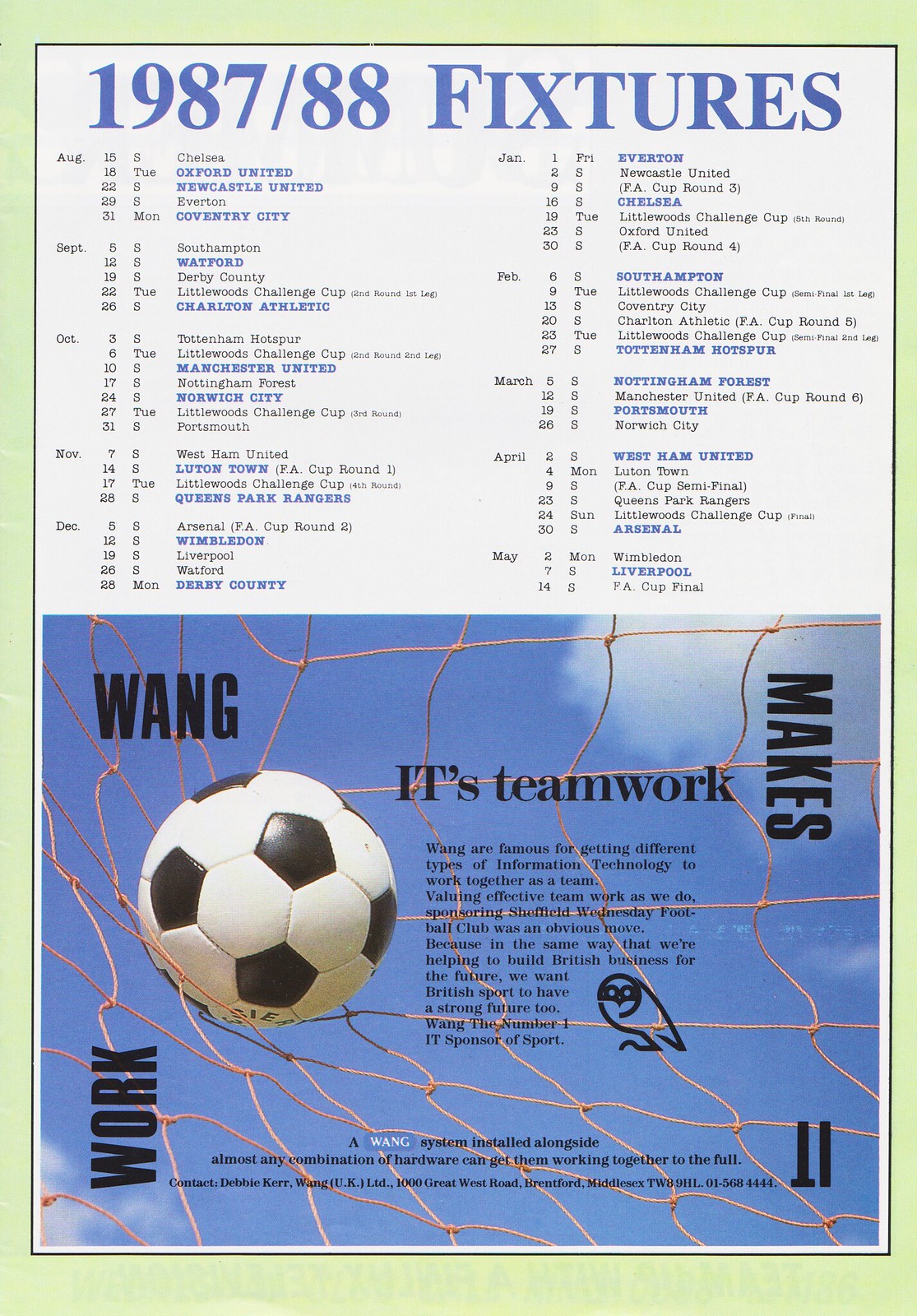This image is a detailed 1987-88 fixtures poster for a soccer team, showcasing a comprehensive schedule and promotional content. The top half of the poster features a white background with blue print listing calendar dates arranged from August to May, detailing the cities where matches will be held, including Oxford, Newcastle, Coventry, Watford, Manchester, Luton, Wimbledon, Derry, Everton, Chelsea, Southampton, Tottenham, Portsmouth, West Ham, Arsenal, and Liverpool. This section serves as the team's schedule.

The lower half of the poster combines imagery and text, with a green background and prominent blue lettering. It includes a detailed advertisement proclaiming, "Work Wang Makes," highlighting the significance of teamwork. A soccer ball is shown in a net, symbolizing the importance of collaboration. Additionally, there is a small owl logo and fine print that promotes Wang's technology integration services, emphasizing their role as a major sponsor of Sheffield Wednesday Football Club. The poster is framed by a black border and ends with contact information for Debbie Kerr at Wang UK, LTD, located at 1000 Great West Road, Brentford, Middlesex, TW89HL, along with the phone number 01-568-4444.